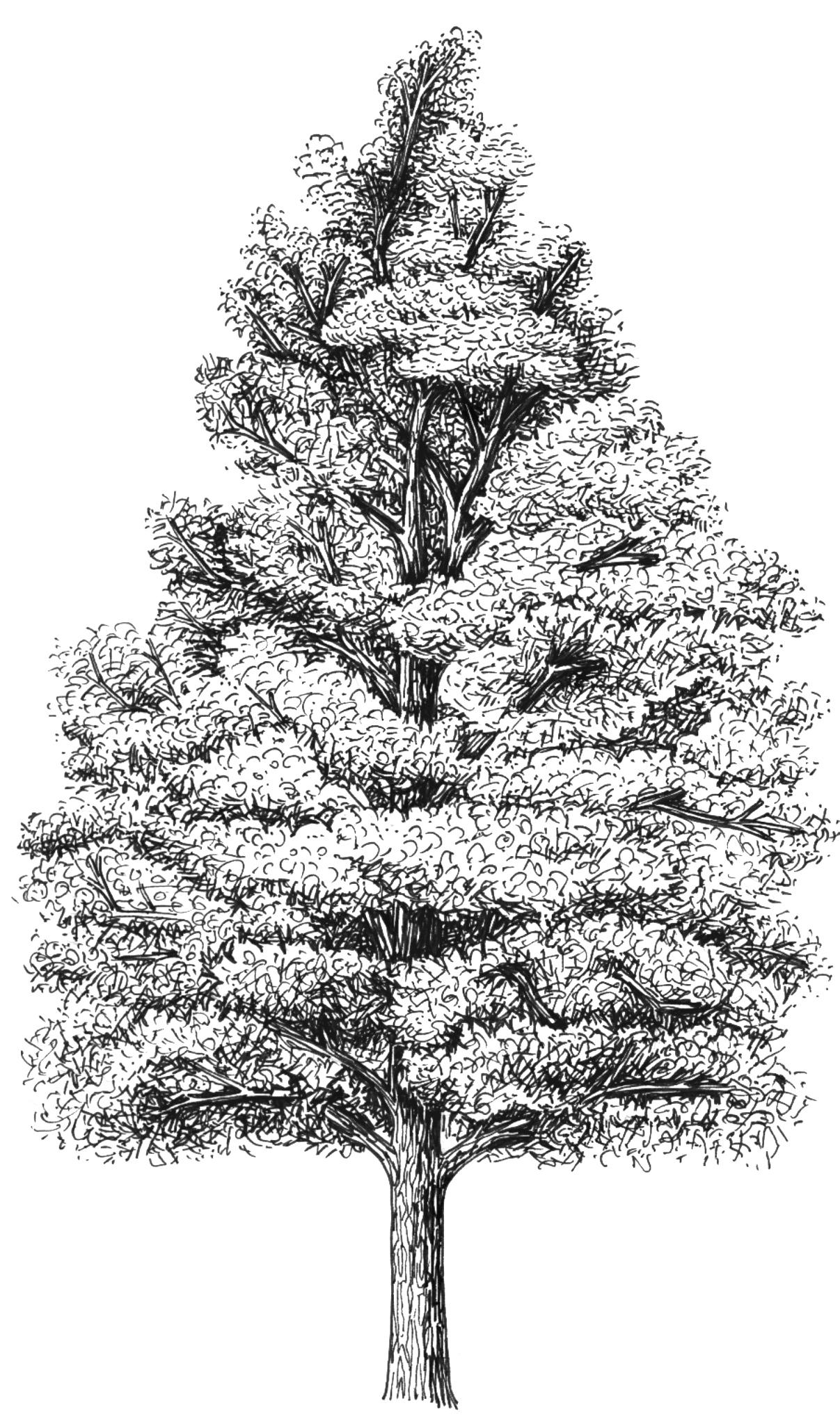This black and white hand-drawn sketch features a tall, robust tree that occupies the entire image. The scene starts at the base of the trunk, which appears partially cut off at the bottom, and extends upward to reveal the full extent of the tree. The trunk is depicted with significant detail, showing its narrow but sturdy nature, and it runs centrally up through the tree, with numerous branches spreading out from it. The tree appears lush and leafy, although the leaf detail is minimal compared to the trunk, resulting in a fluffy and wide appearance reminiscent of an evergreen or Christmas tree. The background is completely white, devoid of any additional elements, emphasizing the tree's prominence. The sketch employs varying shadings of black and white to define the trunk and denser foliage at the top, with sparser sections visible in the upper center. Despite its stylistic simplicity, the tree exudes a strong, lively presence within the image.